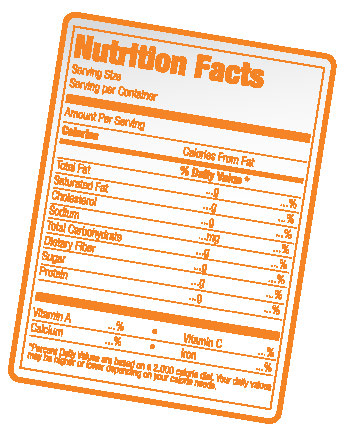The image depicts a Nutrition Facts label set against a stark white background, causing the edges of the image to blend in seamlessly. The label is slightly tilted, with the bottom right corner appearing closer to the viewer while the top left corner tilts upwards. The label itself is prominently bordered with a thick, vibrant orange line, and an additional thinner orange line inside it, encompassing the entire panel.

At the top of the label, the words "Nutrition Facts" are printed in bold orange text. Below this title, standard nutritional categories are listed, such as serving size, servings per container, amounts per serving, calories, calories from fat, and daily values. The nutritional entries include total fat, saturated fat, cholesterol, sodium, total carbohydrate, dietary fiber, sugars, protein, vitamin A, calcium, and iron. Notably, all these categories lack specific numerical data, making the label appear blank and uninformative in terms of actual nutrient content.

A small star at the bottom alludes to the common dietary guideline of a 2,000 calorie diet but does not offer further context or information about the food product itself. Overall, the image represents a generic, incomplete Nutrition Facts label without any personalized specifics for a particular item.